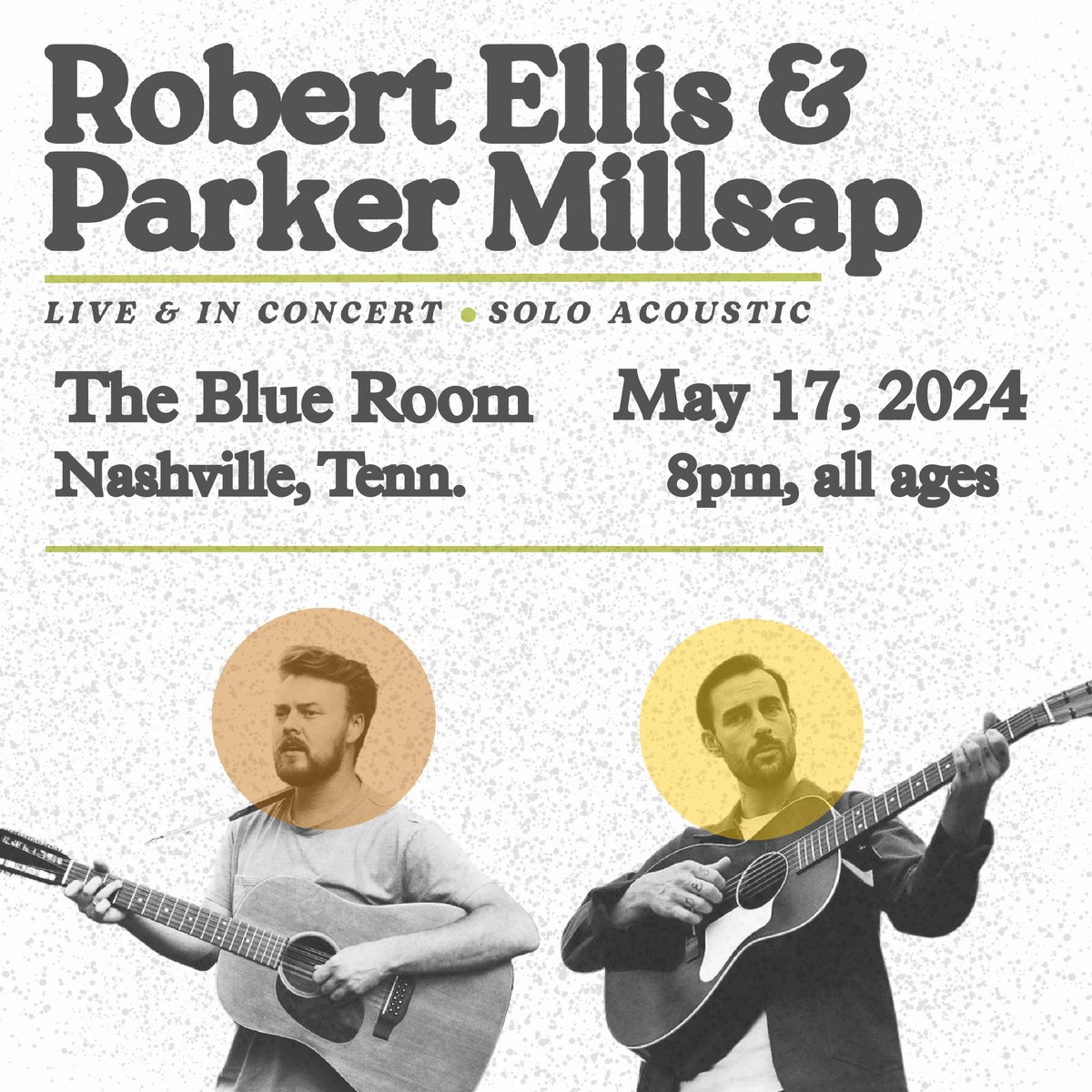The image is a concert advertisement that evokes a vintage feel with its muted colors. The background is white, sprinkled with faint gray specks. At the top left, in large black letters, the names "Robert Ellis and Parker Millsap" are prominently displayed, underlined by a thin green horizontal line. Below this, in black text, it reads "Live and In Concert, Solo Acoustic." Further down, the details "The Blue Room, Nashville, Tennessee, May 17, 2024, 8 p.m., All Ages" are listed in black. 

The lower part of the poster features two side-by-side images of the performers, each playing an acoustic guitar. The man on the left has short brown hair, a mustache, and a beard, and is wearing a short-sleeved, light-colored shirt. His face is framed by a pinkish circle, and he holds a lighter-colored wood guitar. The performer on the right, dressed in a dark-colored black jacket, has darker brown hair and also sports a mustache and beard. His guitar is black, and his face is encircled by a yellow round outline.